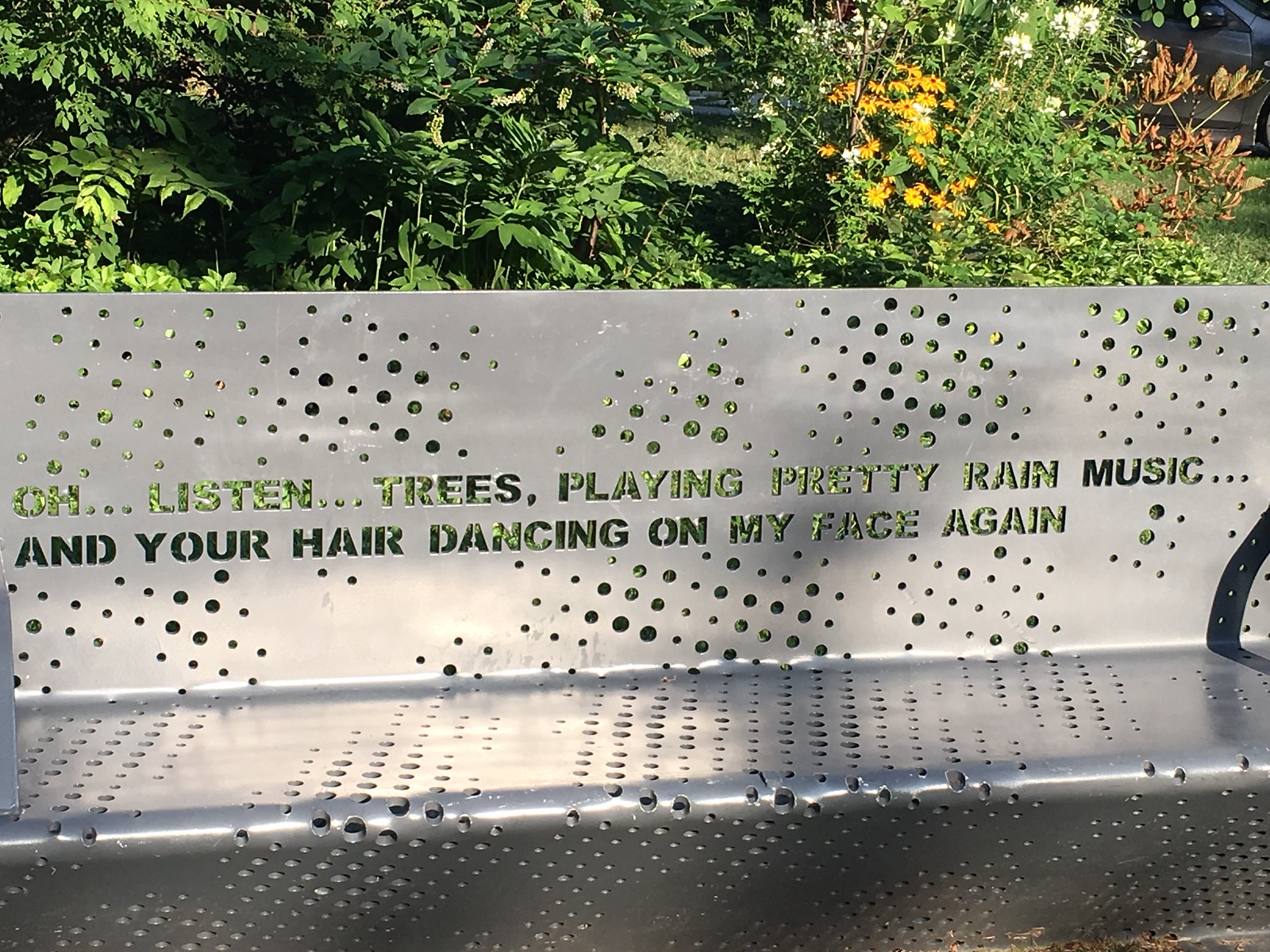This photo features a detailed and shiny grey metal bench, designed with numerous small holes punched throughout its surface. The backrest of the bench prominently displays an inspiring text that has been intricately cut out of the metal: "oh... listen... trees playing pretty rain music... and your hair dancing on my face again." Behind this artistically designed bench, a lush garden of dark green foliage and vibrant flowers is visible, with splashes of yellow and white petals bringing color to the scene. To the right, some brown leaves can be seen, just beyond the edges of the garden, and the top right corner of the image includes a glimpse of a vehicle. This blend of natural beauty and thoughtful craftsmanship creates a peaceful, contemplative atmosphere.